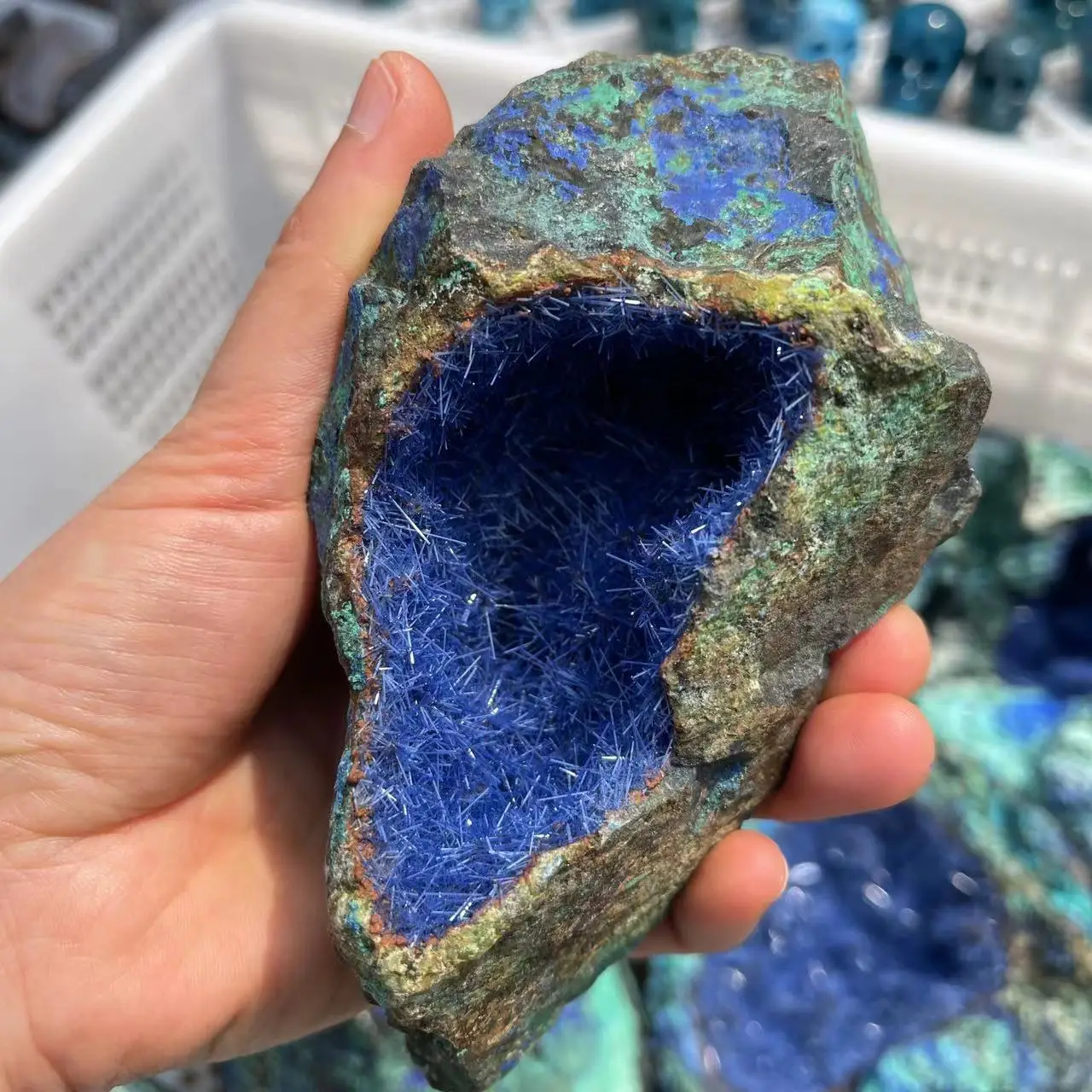In this vertical rectangular photograph, a person is holding a stone closely resembling a geode in their left hand, with their thumb and three fingers visible gripping its sides, as the palm subtly peeks through. The exterior of the stone exhibits a rugged gray surface tinged with hues of blue, purple, and green, along with patches of tan. It uniquely mimics the shape of a human heart. The more compelling feature lies inside the stone: it has a hollow cavity densely packed with dazzling, very small blue crystals that resemble cotton or fiberglass strands. In the background, there is a white container filled with similar stones and small, blue-gray-and-purple miniature skull figurines scattered around the top corners. This setting, complemented by the stark white trays holding various rocks, creates an intriguing contrast to the vibrant and intricate details of the geode being showcased.